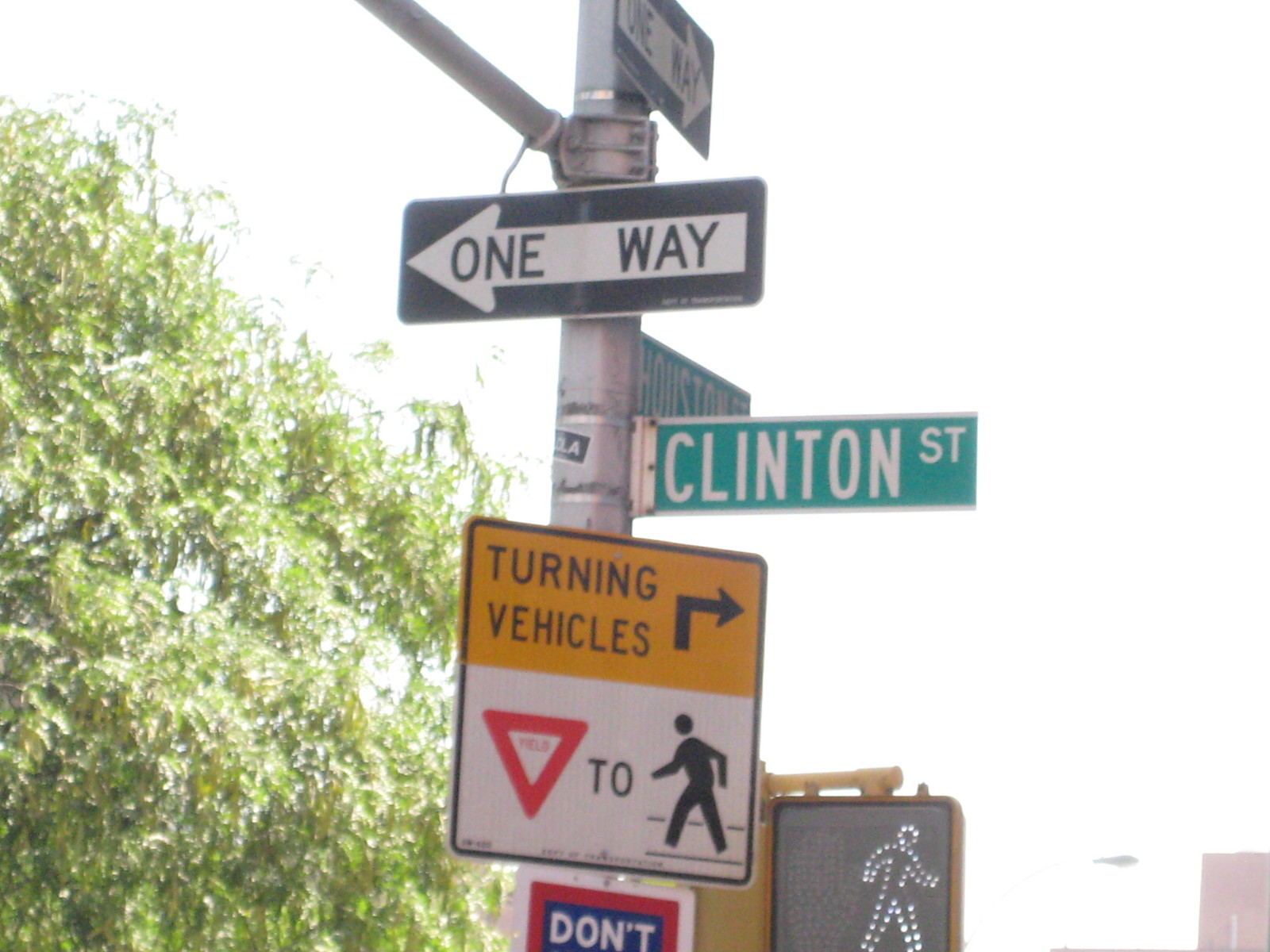This photograph, taken outdoors during the day, captures a detailed view of a metal street pole adorned with multiple street signs. Dominating the left side is a tree whose foliage stretches up from the bottom left to the top left corner. The right-hand side of the image features a white sky. Central to the image, the pole holds various signs arranged vertically. At the top is a rectangular One Way sign with a black background and white text and arrow pointing left. Below it, there's another One Way sign pointing to the right. Descending the pole, the first green street sign indicates Houston Street, directed to the right. Adjacent to it is another green sign for Clinton Street with white lettering. Further down, there's a yellow and white square sign stating "Turning Vehicles" with a right arrow, and below it, a Yield sign that instructs drivers to yield to pedestrians, illustrated with symbols. The lowest sign on the pole is a digital crosswalk sign displaying a lit-up walking person next to the word "Don't." To the left of the pole, lush green leaves from the tree add to the natural element of this urban scene.